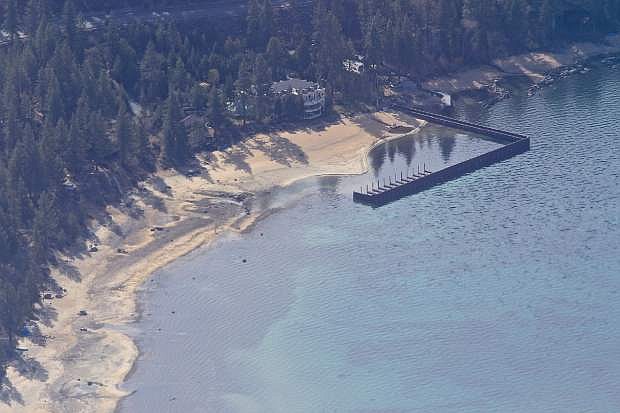An aerial view of a coastline, possibly along the ocean or an expansive lake, reveals a peaceful and heavily forested area dominated by tall evergreen trees. The picture, though grainy, showcases a sandy beach that borders the lush forest. In the middle of the image, there is a prominent L-shaped pier, which extends straight out into the bluish-green water before bending at a 90-degree angle. This water appears somewhat murky, indicating it might not be a tropical location, possibly placing it on an east coast shoreline.

Center stage on the coastline is a sizable building, presumably a house or a resort, nestled in a secluded nook of the beach. This structure stands out with its flat roof, three stories, and balconies, hinting at a private, possibly luxurious property. Despite the warm and sunny weather, the scene is devoid of people, with nobody visible on the beach or in the water.